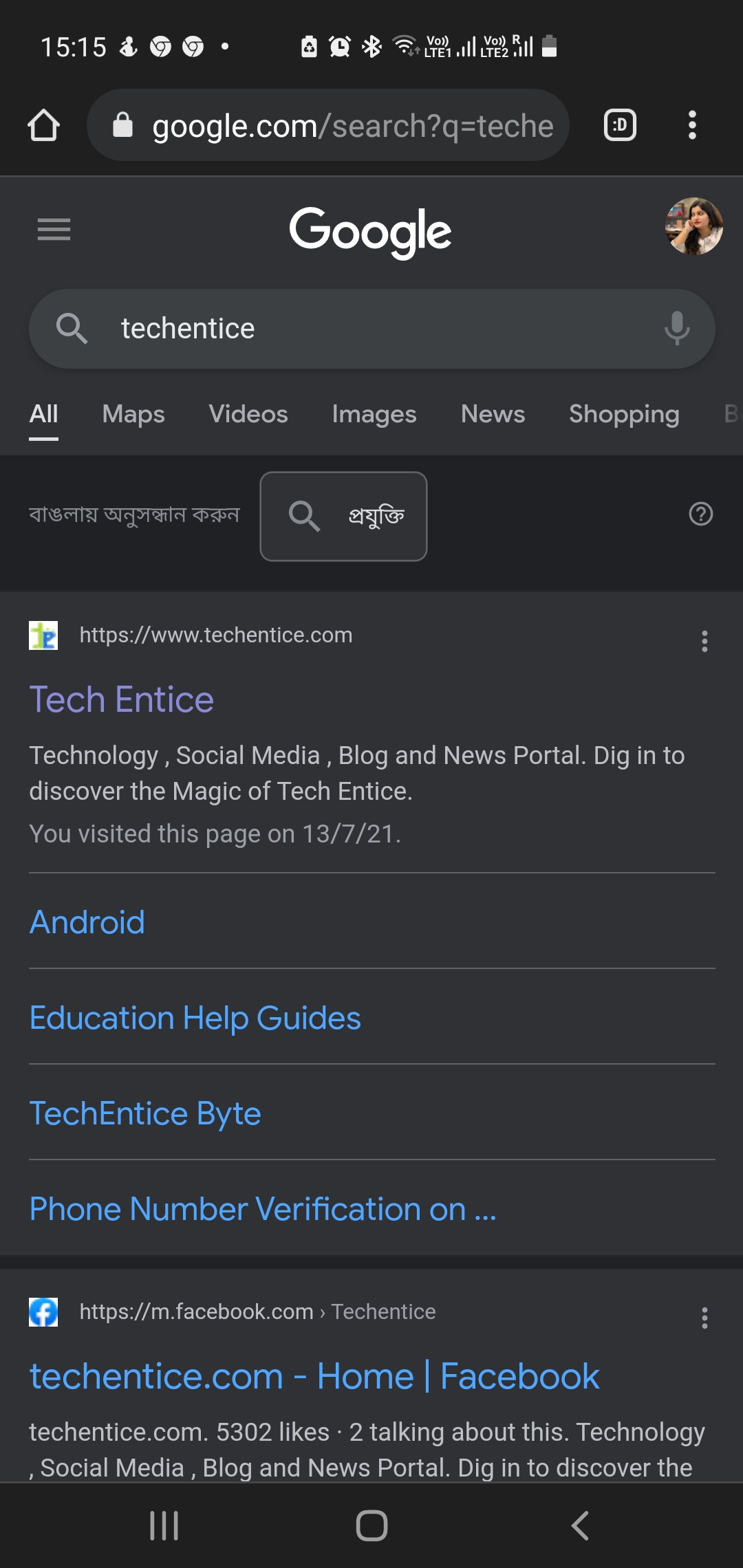The image features a predominantly black background. At the top, there is a segment displaying various icons and symbols. Starting from the left, we see an icon resembling “Thomas 15:15" with a white, running silhouette of a person, likely an app icon. Adjacent to that are two white circles that appear to be volleyball icons, followed by another smaller white circle, possibly signifying notifications. Next, there's a white battery icon and a symbol that looks like two triangles and two lines, whose meaning is unclear. Further along, there is a Wi-Fi signal icon in white and the text "VOLTE" mostly in white, followed by "OLTE2."

Below this section, there is a prominent white silhouette outline of a house. 

The central area of the image is occupied by a web browser interface with an oval-shaped search bar containing "google.com/search?q=TECHENTICE" in white and gray text. Beneath this, in bold white text, is an orange underlined search term "TECHENTICE." Directly below, in gray text, are options such as "Maps," "Videos," "Images," "News," "Shopping," and some text in Hindi.

Continuing down, the image displays the text "Tech Entice" in purple, alongside descriptions like "technology," "social media," "blog news portal," and a tagline "dig into discover the magic of Tech Entice." It also indicates that the page was visited on "13/7/21."

Further below, in blue text, are links labeled "Android," "education," "help guys," "Entice," "byte," "phone number verification," and "Tech Entice - home Facebook."

This detailed description captures the elements and structure of the displayed webpage in the image.